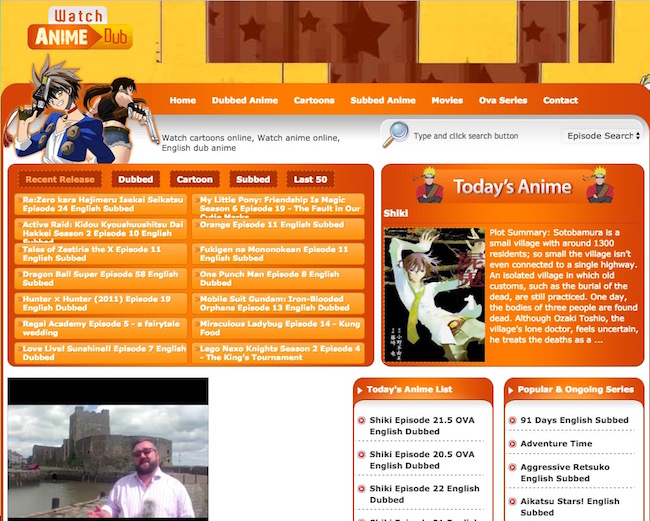The image depicts a webpage from the site 'WatchAnimeDub', displaying various navigation links and anime content. The header section includes links to 'Home', 'Dubbed Anime', 'Cartoons', 'Movies', 'Over The Air Series', and 'Contacts'. The site promotes an array of English-dubbed anime, listing popular series and recent releases.

Prominently featured are series like "Re:Zero", "Active Raid", "Tales of Zestiria the X" (Episode 11), "Dragon Ball Super" (Episode 58), and "Hunter x Hunter (2011)" (Episode 19), all labeled as English dubbed. Additional mentions include "Regal Academy" (Episode 5: A Fairytale Wedding), "Love Live! Sunshine!!" (Episode 7, English dubbed), and "My Little Pony: Friendship is Magic".

The page also highlights a "Today's Anime" selection, featuring "Shiki" with a brief plot summary that describes the setting in Sotobamura, a small village with approximately 1,300 residents, noted for its isolation and lack of highway connectivity.

The design employs a color scheme of yellow, orange, and white, with black text for readability.